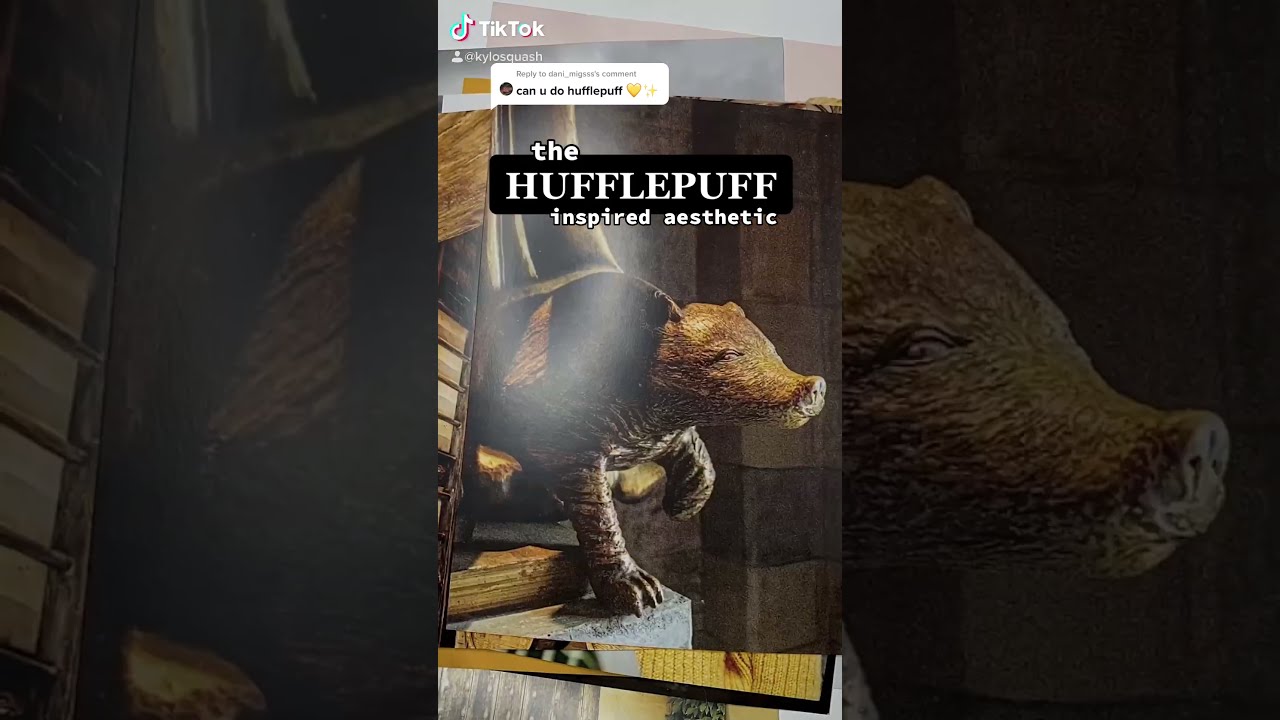This image, a vertically aligned screenshot from a TikTok video, captures a detailed and whimsical scene. Displaying the TikTok logo and handle in the upper left corner, the main focus is a bronze or brownish statue of a badger, expertly crafted or carved to exude a lifelike presence. The badger is depicted mid-stride, with its right front foot placed forward and its left front foot lifted, emerging from a small hutch or burrow. This gives a dynamic sense of movement as if the badger is stepping into the viewer's space. The background behind the figure is a complementary brownish hue.

Overlaying the image, there is a prominent title in a black bar with white text, in an uppercase serif font, reading "HUFFLEPUFF," accompanied by a second line below in lowercase white letters, "inspired aesthetic." At the very top, a screen-captured comment features the question, "can you do Hufflepuff?" followed by a yellow heart and star emojis, creating an intriguing prompt that inspired the content of the video. The detailed craftsmanship of the badger and the themed textual overlays contribute to the overall enchanting and magical aesthetic, resonating with the Hufflepuff house from the Harry Potter series.